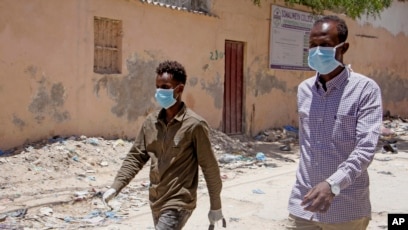The image depicts two Black men walking leftward on a dirty and run-down dirt street, likely in a village in Africa. They are both wearing blue masks that cover their nose, mouth, and part of their neck. The man on the right is slightly shorter, has a receding hairline, and is gloveless, dressed in a purple and white striped long-sleeve shirt and tan pants. His left arm is extended in front of him, and he has a watch on his wrist. The man on the left, appearing closer to the camera, is similarly masked, wearing white gloves, a green button-down shirt, and jeans, carrying something in his left hand. Both men have short, cropped dark hair.

In the background, there's a weathered and deteriorating tan building running the length of the image, with a red wooden door in the center and a boarded-up window to the right. To the left of the door, a white sign with unreadable purple lettering is mounted. The adobe-like structure has patches of brown and gray where the paint has worn off, adding to its dilapidated appearance. The ground is littered with rubble, stones, and garbage, evoking a sense of neglect. At the bottom right corner of the image, the letters "AP" in white capitals are visible within a black box, indicating it is an Associated Press photograph. The overall scene is one of decay and hardship, contextualizing the men's journey through this challenging environment.